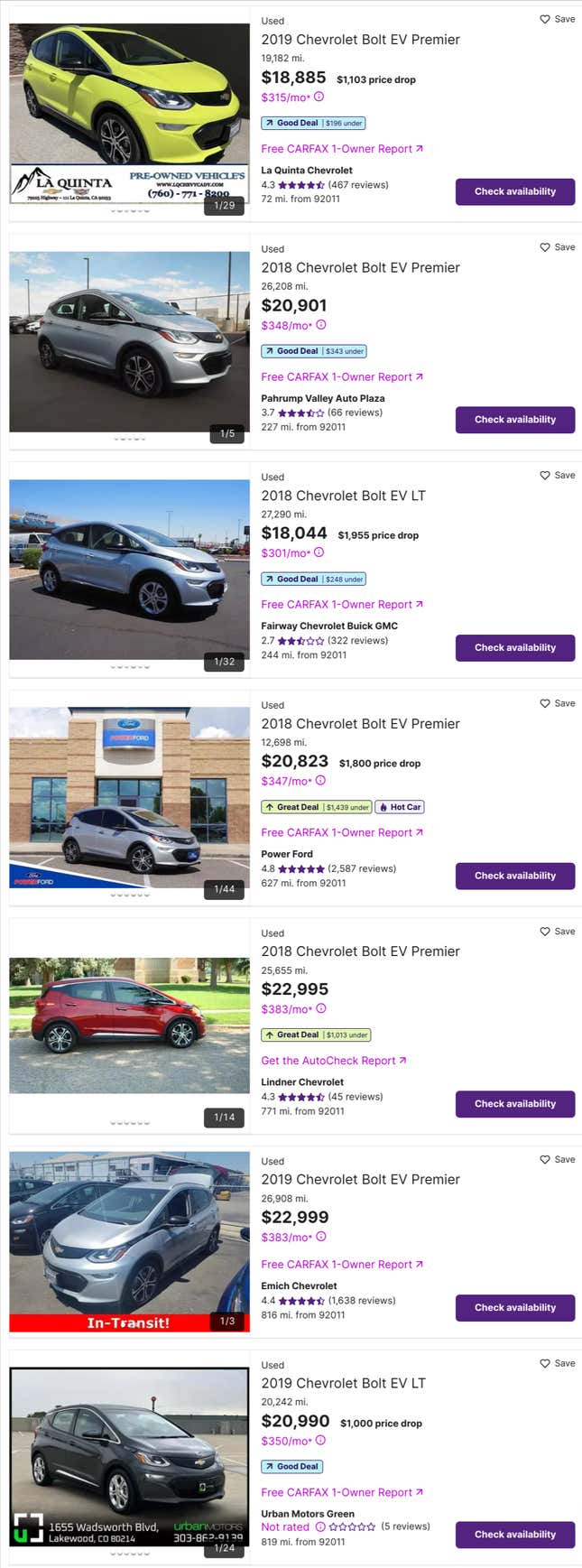This image showcases an entire page of used car listings, specifically for Chevrolet Bolt EVs. All vehicles listed are from the years 2018 and 2019. The prices of these cars range from approximately $18,000 to $23,000, varying based on mileage and condition. The listings feature several color options including neon green, silver, bluish-silver, red, and black. Each car listing includes a purple "Check Availability" button, and it appears that free Carfax reports are available for all vehicles.